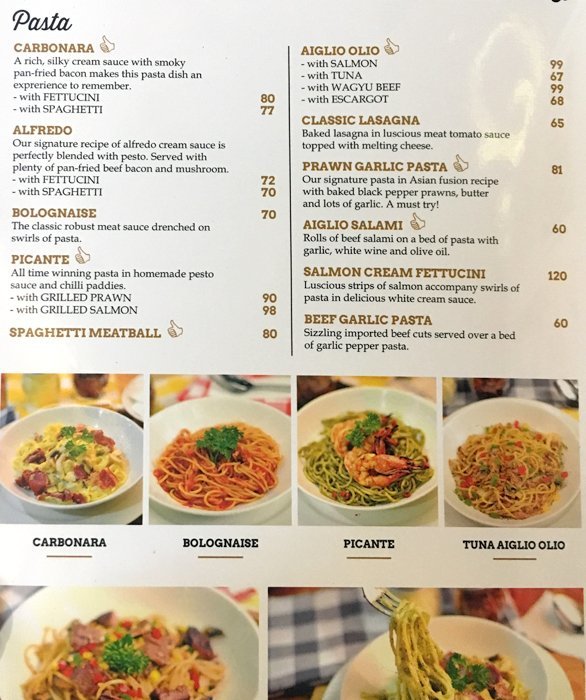The image is a tall, rectangular menu page with a white background, featuring a black cursive title "Pasta" in the top left corner. The menu is divided into two columns at the top, separated by a black line. In the left column, menu items are listed in gold, all capital letters: Carbonara, Alfredo, Bolognese, Picante, Spaghetti Meatball. The right column lists: Aglio e Olio, Classic Lasagna, Prawn Garlic Pasta, Aglio Salami, Salmon Cream Fettuccine, Beef Garlic Pasta. Each item is accompanied by a description and price. Below the columns, there are four square images of pasta dishes labeled in black font: Carbonara, Bolognese, Picante, and Tuna Aglio e Olio. Beneath these are two more images of pasta dishes, partially visible.